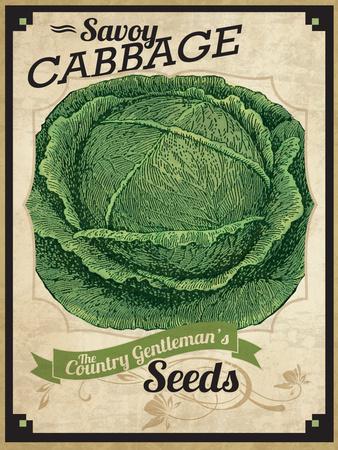The image depicts the cover of a vintage seed packet for "Savoy Cabbage." The overall design features a beige background, adorned with a subtle tan-on-tan texture that adds depth. It is framed by a thin black outline with decorative black squares in each corner, accentuated by tiny green squares. Dominating the center of the packet is a large, green cabbage, illustrated in a semi-old-fashioned style reminiscent of a lithograph, with intricate details highlighting the texture and leaves. 

At the top, in elegant script type, the words "Savoy Cabbage" are prominently displayed. Below, a green banner with beige script type reads "The Country Gentleman's," while beneath it, in black serif type, the word "Seeds" is positioned. The composition gives off a nostalgic feel, suggestive of a professionally made mid-20th-century advertisement, possibly drawing inspiration from Norman Rockwell's era of hand-drawn illustrations.